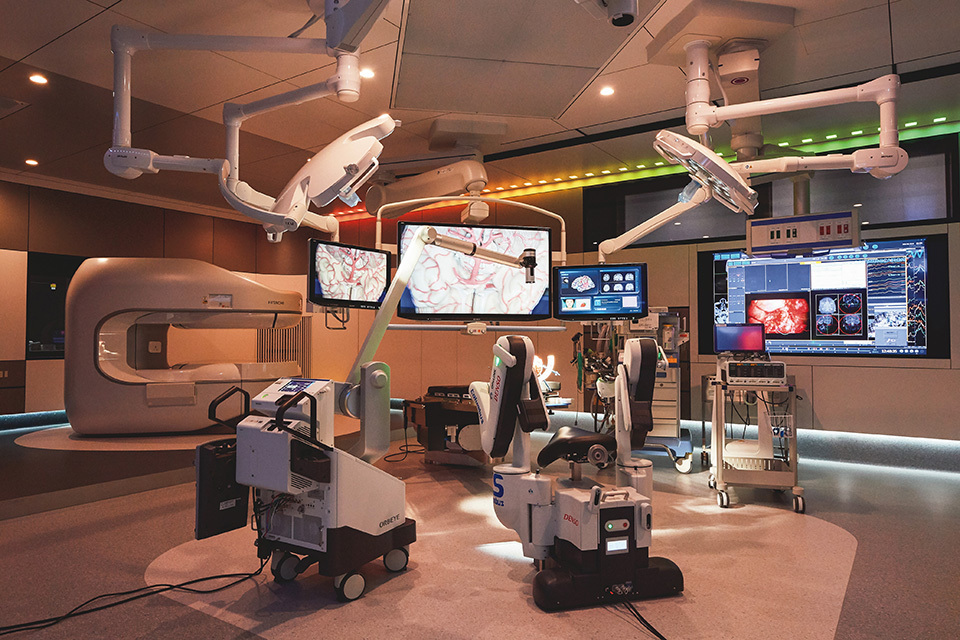The image captures a highly advanced medical facility featuring an operation room. The sleek, modern interior with white walls and gray trim exudes a streamlined aesthetic. On the right side of the back wall, four large TV mounts display intricate details, possibly data about the human brain. Suspended from the ceiling are three flat-screen televisions; the central one is larger, flanked by smaller screens on either side, which showcase detailed images resembling the human brain’s structure.

Flanking these ceiling-mounted televisions are circular operation lights, adding to the array of high-tech equipment. Below these lights are two black-and-white machines, essential for various medical tasks. The room also houses several robotic pieces of equipment, both mounted on wheels and suspended from the ceiling. These robotic arms appear telescopic and versatile, some equipped with cameras, lights, and magnifiers, likely used to handle various medical instruments.

On the left side, there's a white bed positioned under what could be an x-ray or MRI machine, contributing to the room's functionality as a comprehensive medical workspace. The floor, featuring a silver hue, includes a white platform where two robots are evidently stationed, attached to electrical sources. This well-lit, meticulously organized room gives the impression of a cutting-edge medical and scientific robotic laboratory.